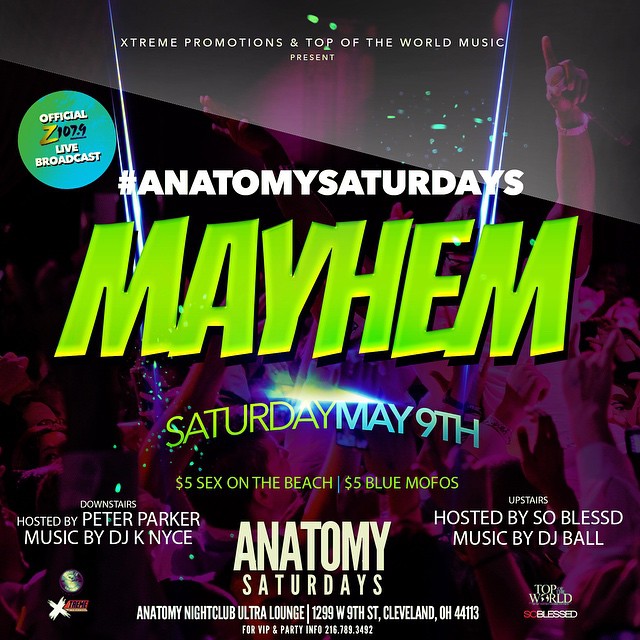The poster for the event features a vibrant and energetic backdrop of pink and black with a crowd of people dancing with their hands in the air, hinting at the lively party atmosphere. At the top, the text "Extreme Promotions and Top of the World Music Present" is written in white. This is followed by the tagline "#AnatomySaturdays" in large white font. Dominating the center of the poster is the word "MAYHEM" in bold, neon green letters, emphasizing the excitement of the event. The date, "Saturday, May 9th" is highlighted in blue, accompanied by drink specials: "$5 Sex on the Beach" and "$5 Blue Mofos." 

At the bottom left, it details "Downstairs hosted by Peter Parker, Music by DJ Gneiss," and on the right, "Upstairs hosted by So Blessed, Music by DJ Ball." Additionally, a blue and green circle with white text in the upper left corner states "Official Z107.9 Live Broadcast." The event venue, "Anatomy Nightclub and Ultra Lounge," is located at 1299 West 9th Street, Cleveland, Ohio 44113. For VIP and party info, a contact number "216-789-3492" is provided. Finally, the poster reiterates "Anatomy Saturdays" in white near the bottom, ensuring the branding is clear and consistent.